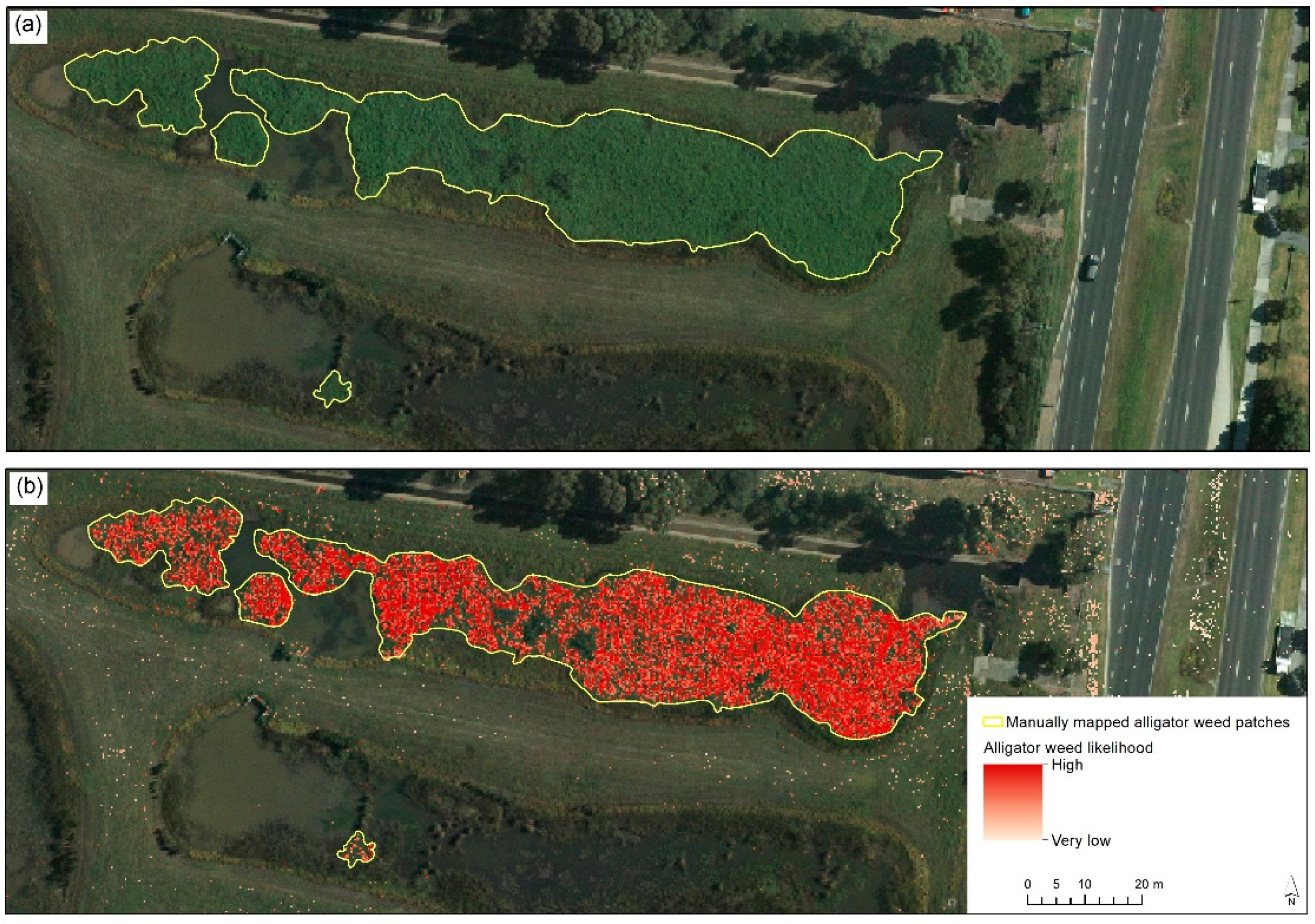This image features two aerial thermal photos labeled A and B, positioned top and bottom, respectively. Both photos exhibit the same land area, with a jagged yellow border outlining a long, narrow pond located centrally within each image. The top photo (A) uses a greenish hue to highlight the area within the border, while the bottom photo (B) employs a spotty red coloration. The red coloration indicates varying degrees of alligator weed likelihood, with deeper reds signifying higher likelihood and pink or white showing very low likelihood. 

In the bottom right corner of the bottom photo, there is a white box with black text explaining the color-coding: "manually mapped alligator weed patches" and "alligator weed likelihood." Additionally, a small arrow pointing north (N) helps orient the viewer. The right side of both photos features visible roads, adding context to the land area shown. This detailed thermal imagery likely serves as a valuable tool for conservationists or land management professionals to assess and compare the presence of alligator weed in the mapped region.